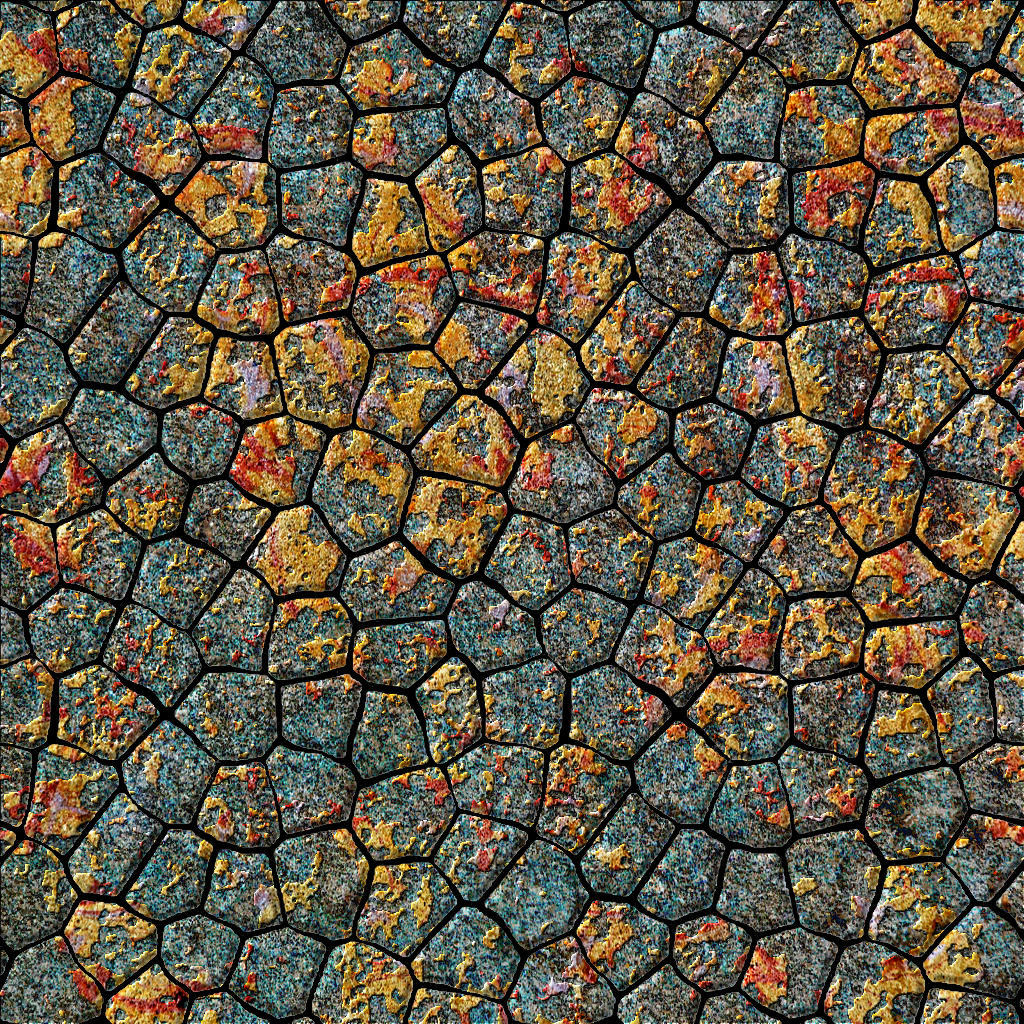The image depicts a visually captivating surface, possibly a floor or wall, composed of an intricate arrangement of interlocking small stones. This mosaic-like pattern features irregular shapes that resemble a honeycomb, with rocks varying in sides and sizes, some being quadrilateral while others have five or six sides. The stones are predominantly gray-blue in color, creating a consistent but varied palette. Notable splotches of red and yellow adorn many of the rocks, reminiscent of dried mustard and ketchup, adding vibrancy and texture to the scene. The meticulous construction suggests an artisan's touch, as the stones fit together seamlessly, showcasing both the natural beauty of the individual rocks and the skill involved in their assembly. Overall, the composition is both complex and aesthetically pleasing, combining natural elements with an artist’s precision.